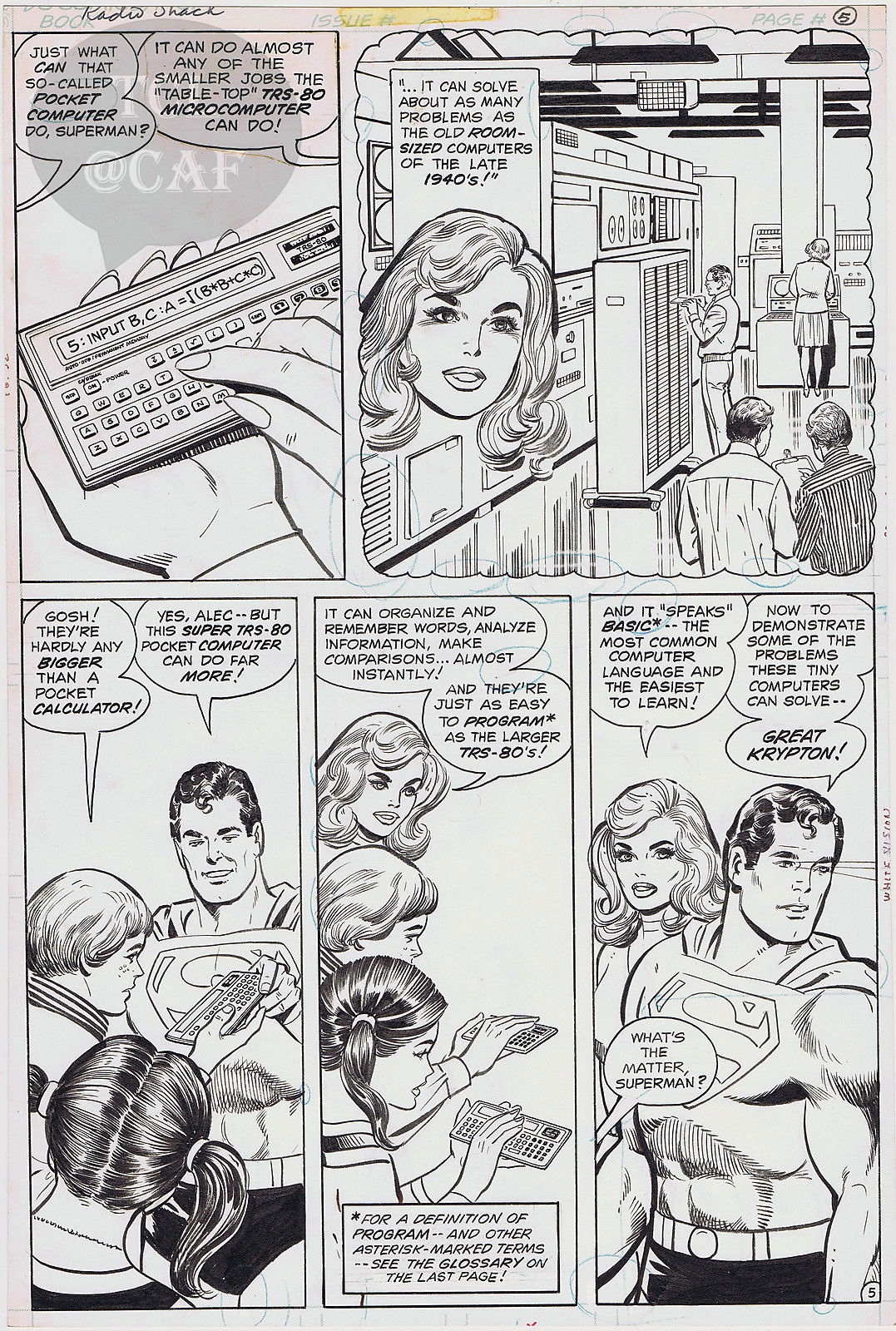This black-and-white comic book page features multiple panels, primarily showcasing Superman and a group of people, including a woman and possibly her children, in a techno-industrial setting with large, old-fashioned computers. The top left panel depicts two hands typing on a device resembling a vintage calculator, with speech bubbles indicating dialogue. The top right panel focuses on a close-up of a woman's face with text above, set against the backdrop of the room with multiple individuals working at computers. In the middle, Superman is seen conversing with a young girl with ponytails and a boy, while another panel features the same girl and boy with the woman instead of Superman. The final panel shows the woman and Superman engaged in discussion, with multiple speech bubbles illustrating the extensive dialogue about problem-solving capabilities compared to mid-20th-century technology. The overall theme suggests a collaborative effort to resolve an issue, with text-heavy dialogue contributing to a classic, detailed comic book aesthetic.